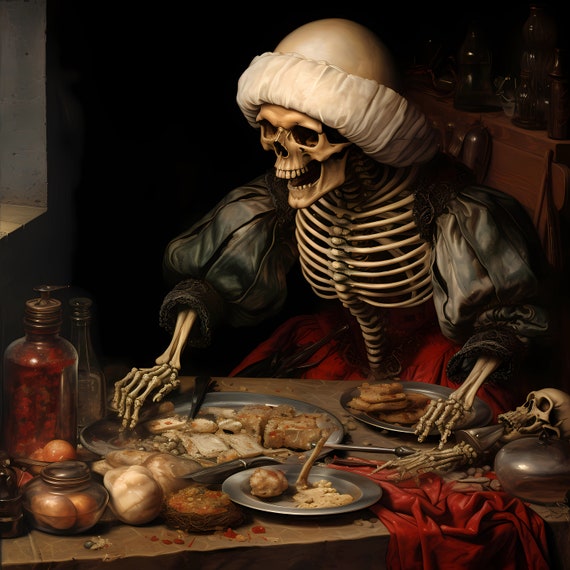The digital artwork features a striking vertical rectangular composition with no border, set against a black background. Dominating the scene is a human skeleton seated at a table, dressed in Middle Ages-inspired attire. The skeleton wears poofy black sleeves and red bottoms, with a white, fluffy bandana wrapped around its skull. Its mouth is agape, suggesting a smile. The skeleton's rib cage and hands are prominently visible, detailed against the dark ensemble.

In the upper left-hand corner, partial light filters through what appears to be a windowsill, while the upper right-hand corner is cluttered with various containers, including tea kettles and glass bottles. The table before the skeleton is laden with an assortment of foods, including meats, vegetables, and onions strewn messily across silver plates. Additionally, the tablecloth is red and hangs off the edge of the brown table. Notably, the scene includes a smaller skeleton head with a silver conical object on the table, alongside a peculiar utensil resembling a skeleton hand.

The combination of these elements – the rich details in the attire, the variety of food items, and the dynamic positioning of the skeletons and objects – creates a vibrant and somewhat macabre tableau, offering a peculiar yet engaging feast for the eyes.